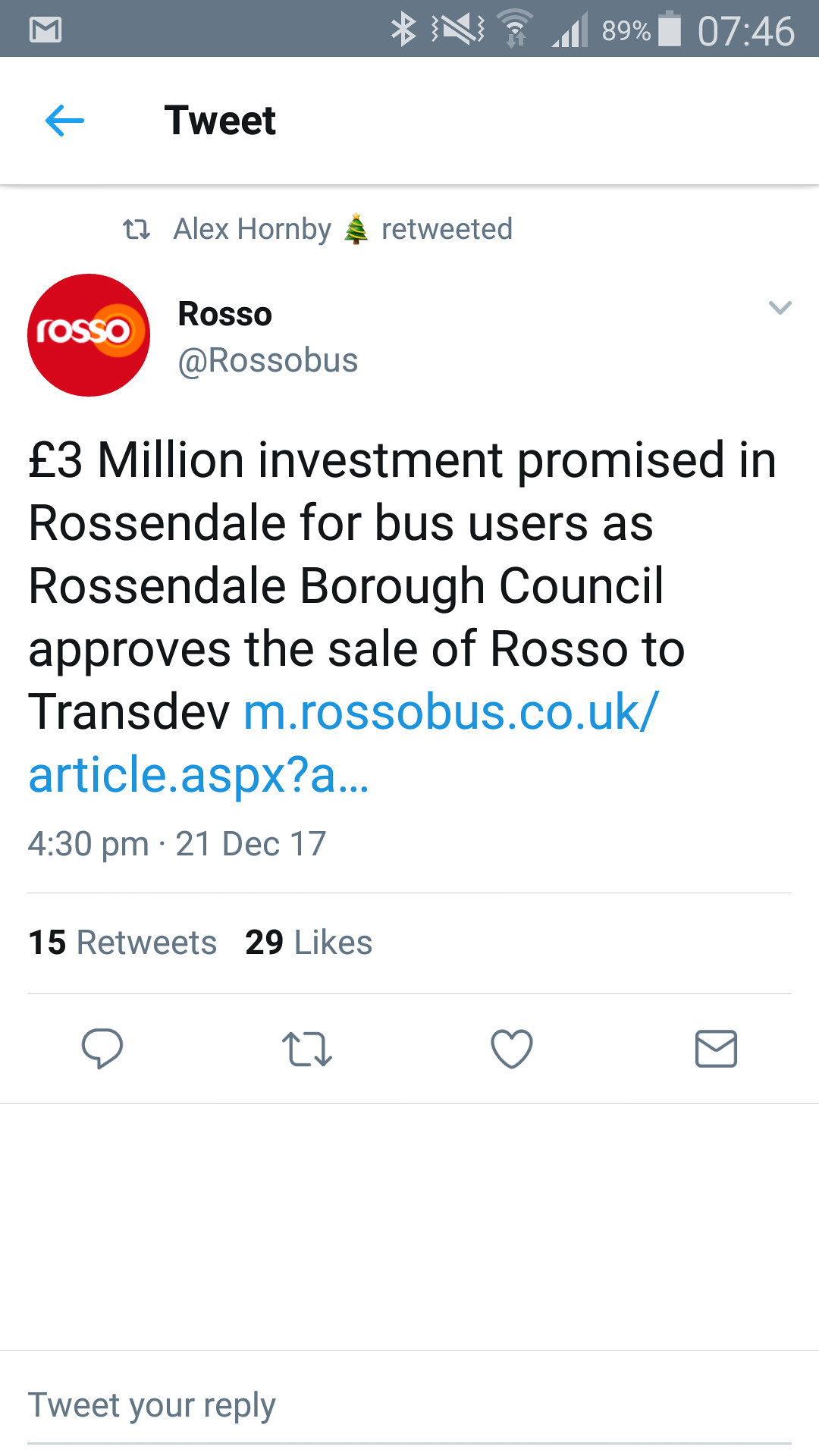The image depicts a tweet viewed on a mobile device, originally posted by Ross Obus and retweeted by Alex Holmby. The tweet announces a £3 million investment in Rossendale's bus services, following Rossendale Borough Council's approval of the sale of Rosso to Transdev. The main text reads: "Three million pound investment promised in Rossendale for bus users as Rossendale Borough Council approves the sale of Rosso to Transdev," accompanied by a clickable link to rossobus.co.uk. The tweet is timestamped at 4:30 PM on December 21st, 2017, and has received 15 retweets and 29 likes. The visual elements include the Rosso logo, which features a red circle with white text and an orange-bordered 'O' in the center. The tweet interface displays the usual interaction buttons for retweeting, replying, and liking, set against a white background on the mobile screen.